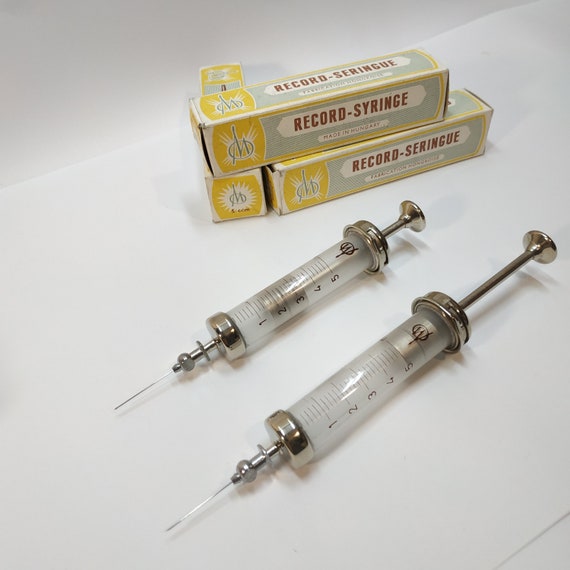A meticulously arranged color photograph features two syringes and three syringe boxes, all set against a pristine white surface. The two syringes are placed diagonally, extending from the upper right to the lower left of the image. Both syringes boast sleek chrome plungers and matching chrome caps. Their barrels are made of a whitish opaque material, marked with measurements from 1 to 5. The needles, crafted from chrome, appear long and razor-sharp. In the backdrop, three vintage-looking syringe boxes are neatly aligned, exuding an air of antiquity. These boxes come in three distinct colors: gold, light gray, and white, each emblazoned with the name "Record Syringe." The overall composition of the photograph captures the juxtaposition of the clinical precision of the syringes with the nostalgic charm of the old boxes.